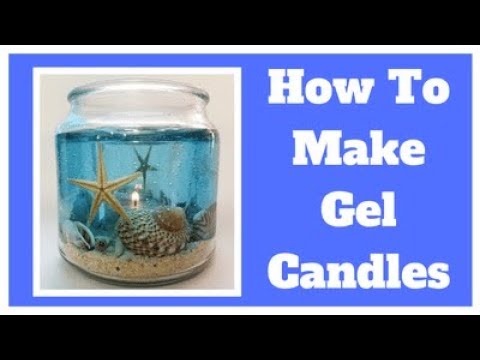The image is a thumbnail from a video tutorial titled "How to Make Gel Candles," with black borders on the top and bottom and a white border around the main subject. Featured prominently is a glass jar, roughly 12 ounces in size, filled with blue gel that mimics water, creating a mini-aquarium effect. The bottom of the jar is layered with sand, speckled to resemble the ocean floor, and dotted with various sea elements—a starfish, seashells, and what looks like a sea urchin shell. The starfish and seashells are positioned against the sides of the jar, making them clearly visible. In the center of this blue gel, there is a lit flame. The jar is designed to look like an underwater scene with its sand and sea life elements encapsulated in a translucent, blue substance, highlighting the candle-making process and final aesthetic.